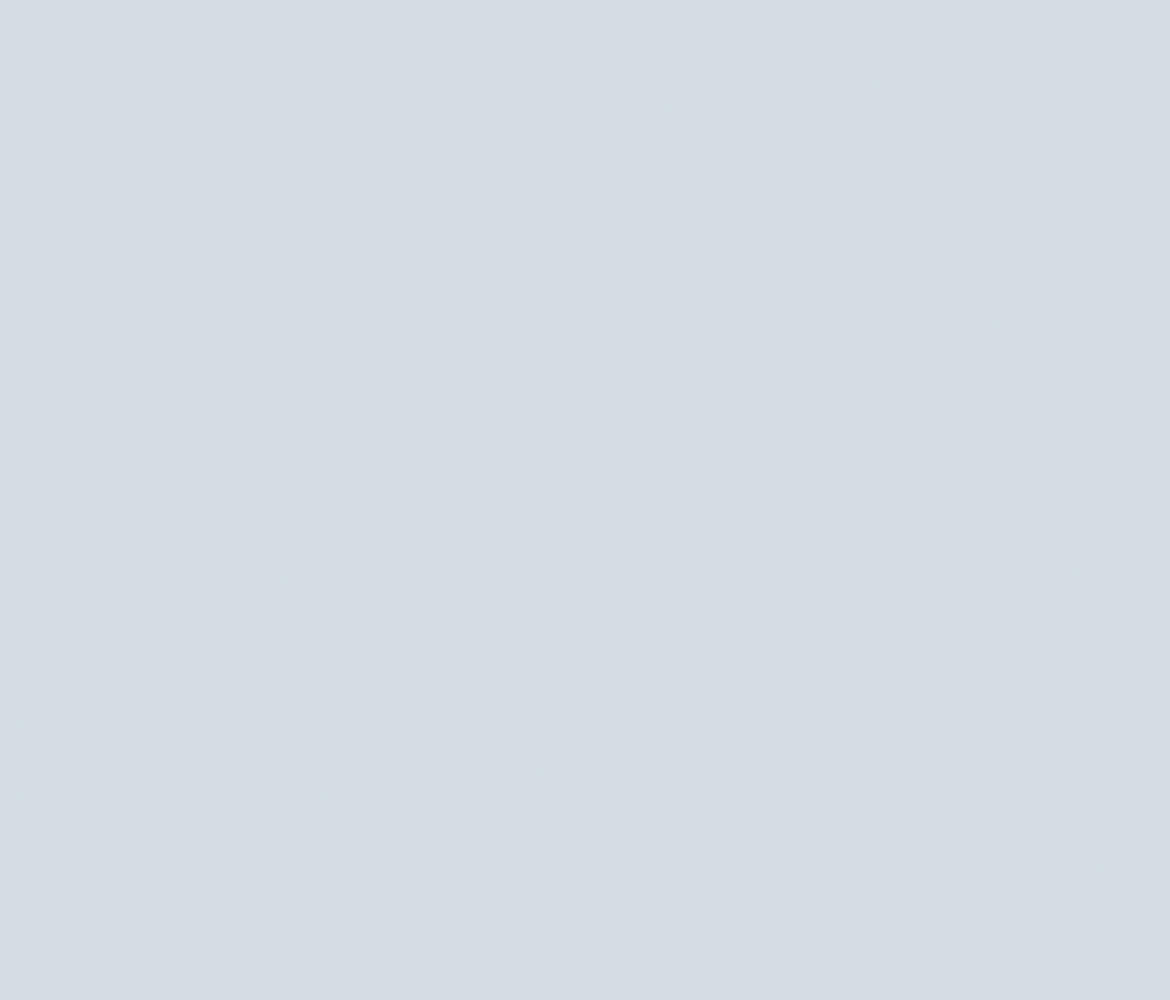Here is the refined and detailed caption:

"A non-existent, square-shaped screenshot is presented with a gray, featureless interior. The image has distinct corners: two on the left and two on the right, and is defined by clear, straight lines running vertically and horizontally along each edge. To the right of this gray square, there is a smaller yellow box containing several questions in black text. These questions prompt the viewer to consider aspects such as the immediate impression of the image, the objects and their counts, text content, object positions, noticeable details, background elements, as well as the style and color of the image. The overall presentation is minimalistic, lacking in style and hues beyond the gray square and the contrasting yellow prompt box."